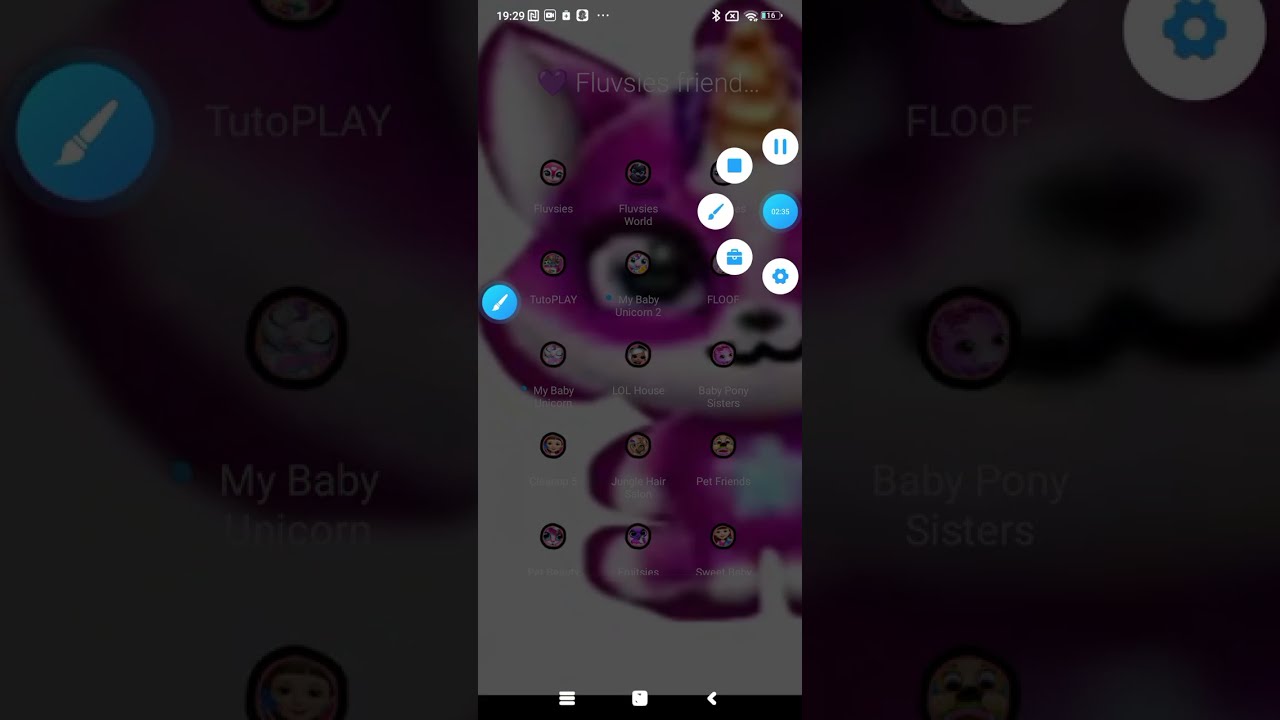The image is a horizontally rectangular digital screenshot, predominantly gray in color. It appears to be the background or screensaver on a device, likely a computer or phone. In the upper left corner, there’s a blue circle icon with a paintbrush, suggestive of a paint or editing application. Next to it, the time is displayed in military format, along with various open icons, indicating a busy or active screen. On the upper right corner, there’s a white circle with a blue gear symbol, possibly for settings.

The background features a series of circular images along the sides, which appear faded and grayed out. These circles are app icons or game images labeled with titles such as "My Baby Unicorn," "Baby Pony Sisters," and "Floof." Dominating the center is a large, vertically oriented image with a light purple background, showcasing a purple and white cartoon creature. The character resembles a baby bear or cat, with distinctive white features including part of its eye, ear, mouth, and tummy. Notably, the creature wears a cap situated between its ears.

Overall, the scene presents an organized yet vibrant digital space, with emphasis on the central cartoon character and surrounded by various game and app icons.